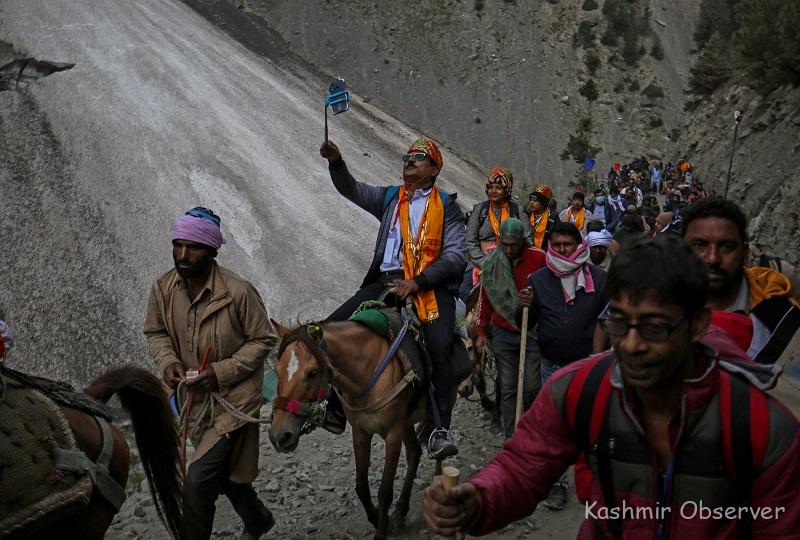The image captures a vibrant and dynamic scene of people traversing a steep, slate-gray rocky mountain path. Most are on foot with walking sticks, while a few are on horseback. The travelers, possibly of Indian or South Asian descent, showcase a variety of colorful attire, including turbans, scarves, and traditional clothing, suggesting cultural diversity. At the bottom right of the image, a man with dark black hair, black glasses, and a backpack uses a walking stick in his left hand. Close by, another man on horseback, adorned with sunglasses, a bright orange scarf, and a red turban, holds a selfie stick to capture the scene behind him. The rocky landscape surrounding them is dotted with sparse green vegetation, and the terrain appears challenging, emphasizing the arduous nature of their journey. Written text at the bottom of the image reads "Kashmir Observer," hinting at a journalistic context, possibly covering a story of migration or a peaceful protest. The image collectively portrays a sense of movement, cultural richness, and resilience amidst a striking geological backdrop.